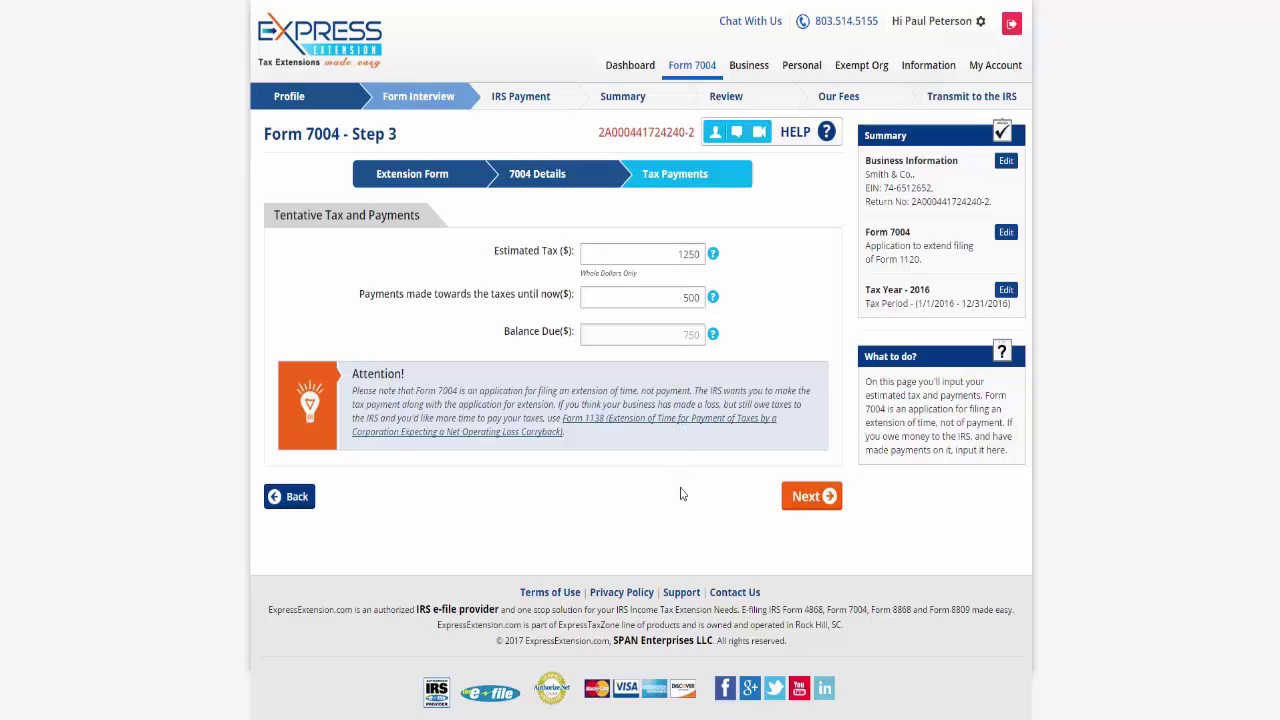**Express Tax Extension Interface:**

At the top of the webpage, the title "Express" prominently highlights that tax extensions are made easy. Positioned at the right-hand corner, users can find a "Chat with Us" support feature. Below that, the user is greeted with "Hi Paul Peterson" next to a gear settings icon that provides access to various options — Profile, Form Interview, IRS Payment, Summary, Review, Fees, and Transmit to IRS — as well as a Help button for additional assistance.

Centrally displayed is the heading "Extension Form" with specific details:
- **Form 7004 Details:** 
  - **Tax Payments:** 
    - **Tentative Tax Payments:**
      - **Estimated Tax:** $1,250
      - **Payments Made Toward Taxes Until Now:** $500
      - **Balance Due:** $750

An important notice is highlighted: "Attention: Please Note, Form 7004 is an application for an extension of filing time, not a payment extension. The IRS expects a tax payment to be made along with the extension application. If your business has incurred a loss but still owes taxes and you require more time to pay, utilize Form 1138 for an extension of time for payment of taxes by a corporation."